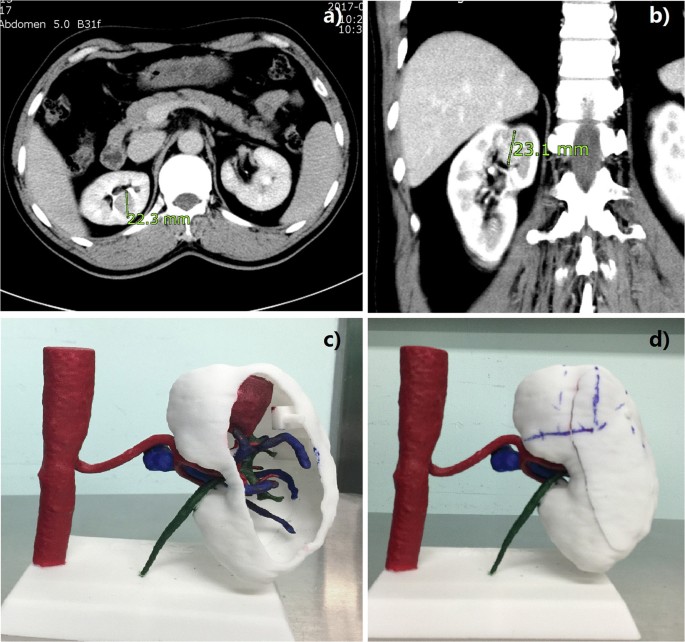The image features a four-panel layout, each labeled A, B, C, and D, which appears to be an illustration for a scientific paper or textbook.

The top left panel (A) displays a black and white scan of an abdomen, likely an ultrasound or X-ray, with visible labels and measurements in green text, indicating sections within the abdominal cavity. Beside it, the top right panel (B) shows another black and white scan, possibly an MRI of the spinal region, marked with numerical measurements.

The bottom left panel (C) showcases a 3D model of what resembles a kidney. This model includes a prominent red stalk emerging from a white base, depicting intricate internal structures with blue and green lines, representing blood vessels or ducts in a cutaway view. Adjacent to it, the bottom right panel (D) presents the same 3D kidney-like model from a different angle, but this time intact without a cutaway, highlighting its external anatomy.

Together, these images provide a comprehensive visual representation of both the internal scans and physical models of relevant anatomical structures, focusing primarily on a section of the abdomen and possibly the kidneys.